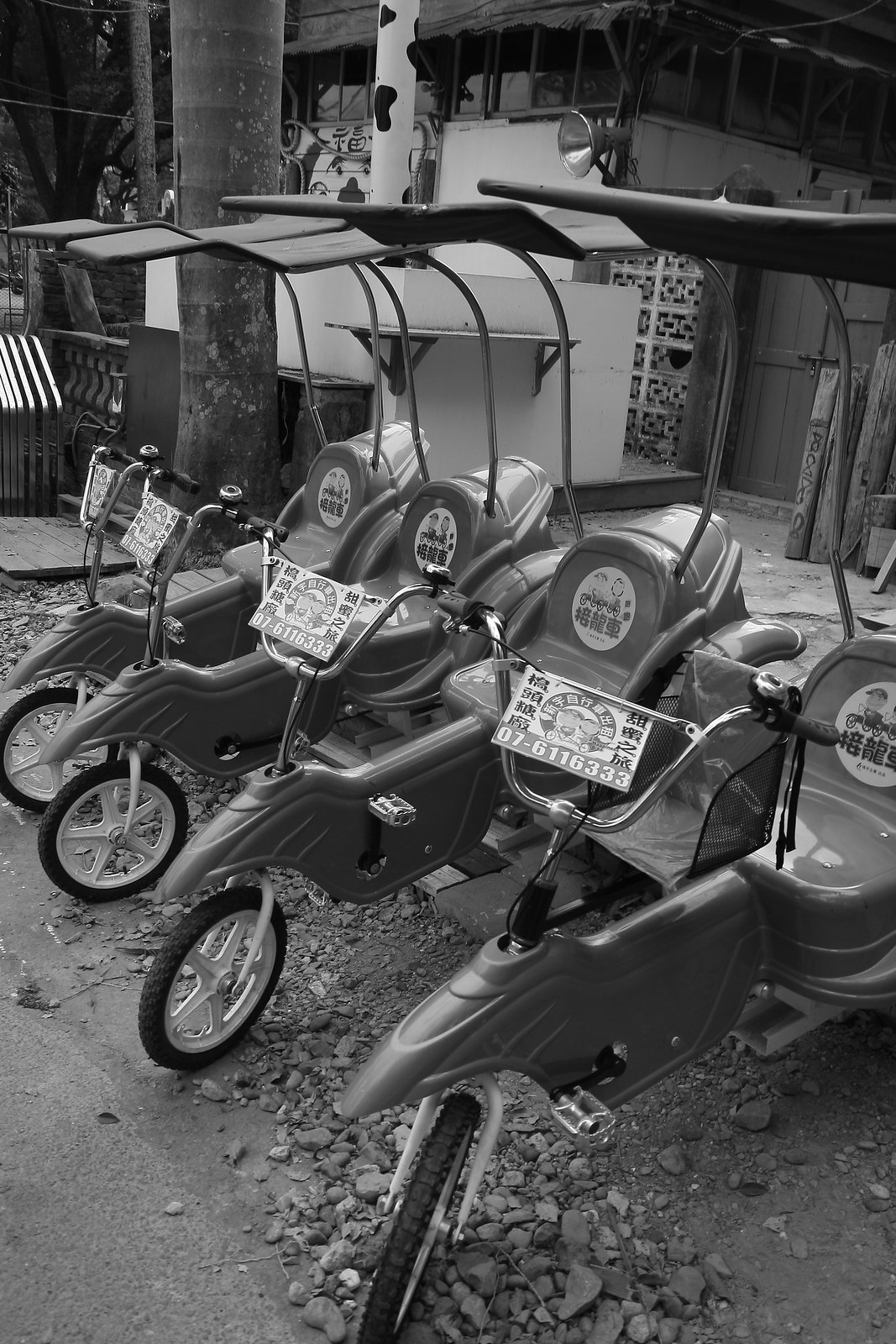This black-and-white portrait-oriented photograph depicts a row of four electric bicycle-like rickshaws, possibly located in a small Asian city, suggested by the non-English characters, potentially Japanese, on stickers attached to the back seats and handlebars. These rickshaws feature plastic bucket seats with black covers and plastic sides along the bike frames. Each rickshaw has a front tire pointed to the left diagonal and bars rising from the back of the bucket seats, supporting small awnings above. The foreground showcases these vehicles lined up from the bottom right corner of the frame and extending away from the viewer. Set on what appears to be a rocky or brick-surfaced road, the background transitions into a diagonal curb leading to a sidewalk. Further back are several tree trunks, one dark and one light with patches, alongside buildings with wooden paneling, glass panels, and some trellis elements. The tight crop leaves ambiguity as to whether the location is a street in a commercial or residential district.